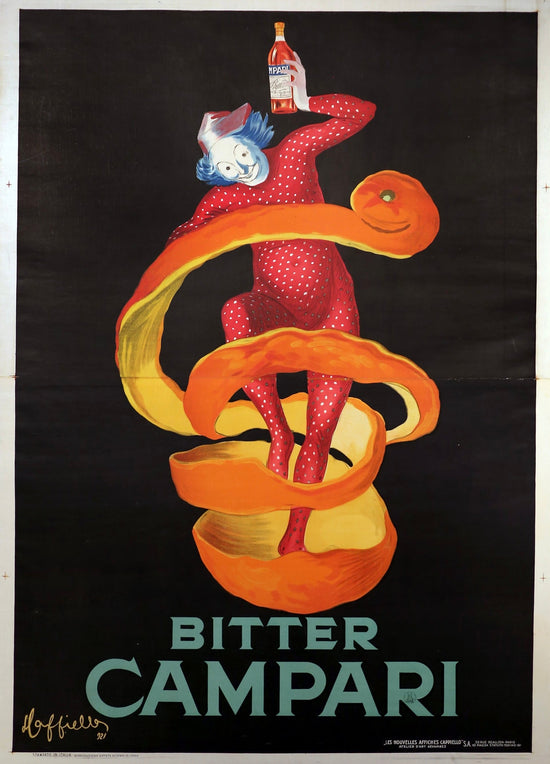This vintage advertisement for Campari features a striking composition set against a black background with an outer gray border. At its center, a circus clown dressed in a red unitard with white polka dots takes the spotlight. The clown's face is painted white, accentuated with large eyes and framed by blue hair that flares out from the sides. A small red cap tops the clown's head. The clown strikes a whimsical pose; its left arm extended outward at the shoulder, bent at the elbow, with the forearm raised near the head to display a bottle of liquor. The bottle, labeled but too small to decipher, is gripped in the clown's left hand.

Adding a playful touch, the clown is encircled by a spiraling peeled orange, creating the illusion that the clown is emerging from this citrus swirl. The peel wraps around the clown's body and creates a base at the bottom. Below this vivid scene, the advertisement's text features bold, vintage-style blue lettering. The first line reads "BITTER," followed by a more prominent "CAMPARI" in capital letters. In the lower left corner of the ad, a handwriting-like signature appears but is too small to read clearly. Similarly, the lower right corner contains white printed text with brand details, also too small to be legible.